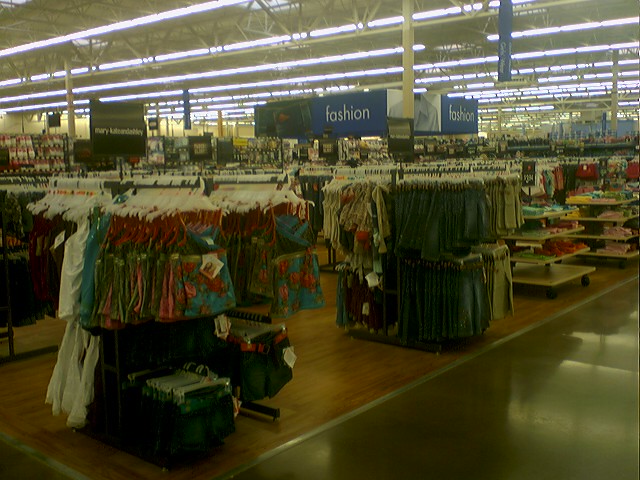The image depicts the interior of a department store, possibly a Walmart, though it lacks the characteristic gold asterisk symbol typically seen in Walmart signage. The store features an open ceiling with visible metal joists and long fluorescent lights hanging from above. The scene is set in the clothing section, specifically labeled "Fashion". The flooring beneath the clothing displays appears to be vinyl planking designed to mimic wood, while the high-traffic walking areas are covered with shiny linoleum for durability. In the foreground, there is a display of multi-colored skorts.